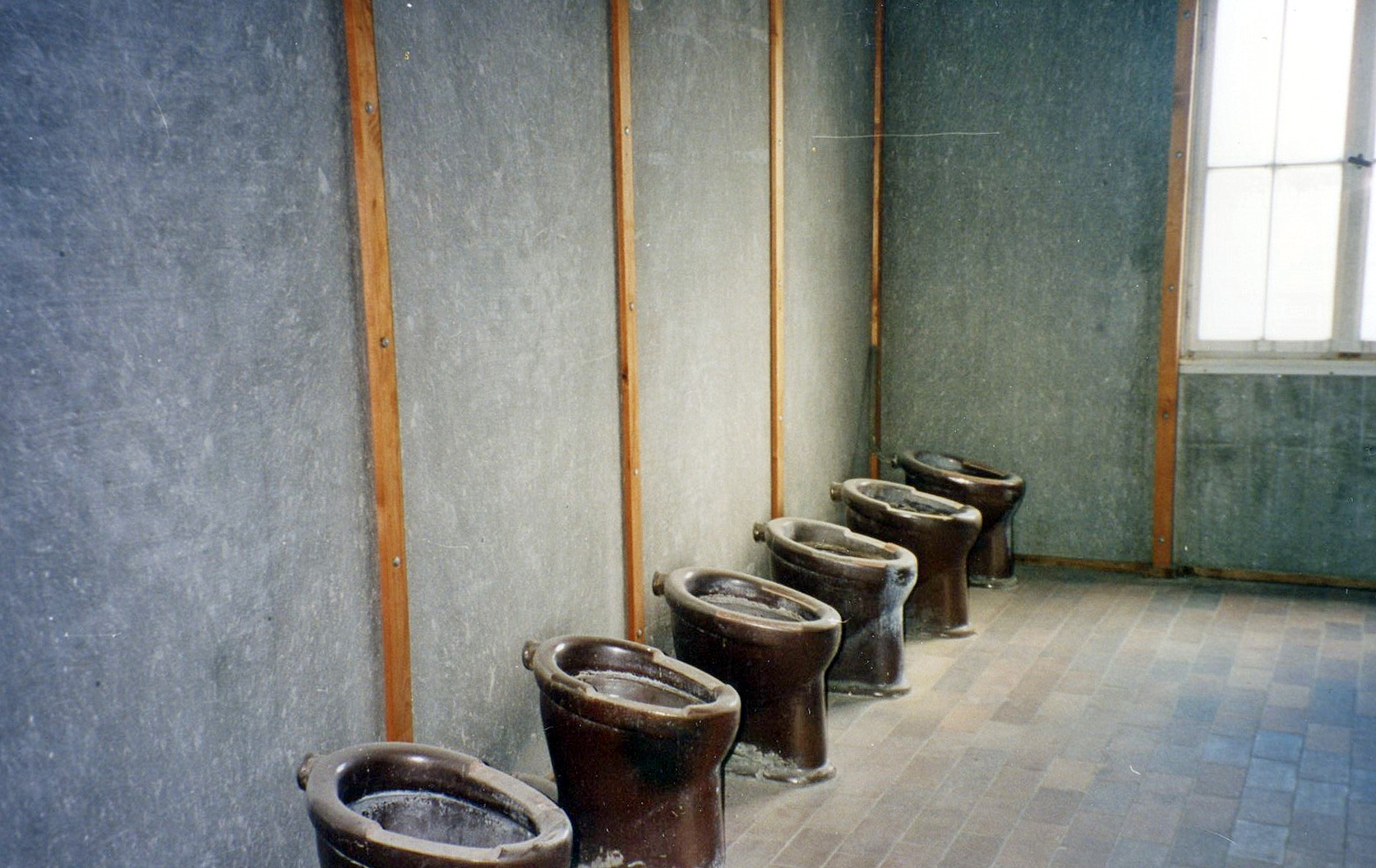In this color photo, we see an unfinished home with a close-up of a plain, patchy gray wall, possibly made of drywall or plaster, intersected by thin, long brown wooden slats running vertically from floor to ceiling. Along the left-hand side of the wall, there are six bare, unconnected toilet installations. These toilets, characterized by their metallic tops with brown, copper-like hues, lack lids and appear dirty and dusty. The bottom portions of the toilets are black metal supports. Sunlight streams in from a window on the right-hand side, indicating it is daytime. The floor appears to be a linoleum designed to mimic cobblestone or brick, comprising various shades of black, light brown, and tan squares, contributing to the unfinished and rudimentary ambiance of the scene.